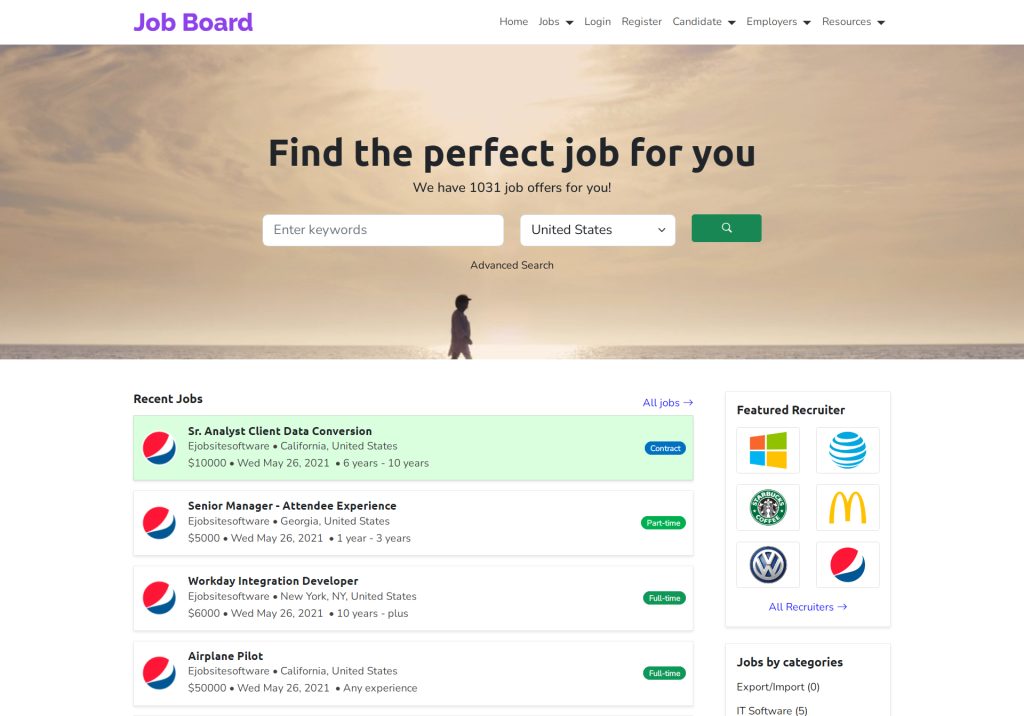This is a screenshot of a job board website. At the top, bold purple text displays "Job Board," accompanied by navigation links to "Home," "Jobs," "Login," "Register," "Candidate," "Employers," and "Resources" on the right.

The main section features a rectangular photograph of a person silhouetted against a grayish-orange sky. Above the image is a headline stating, "Find the perfect job for you," followed by text that reads, "We have 1,031 job offers for you." There is a search bar prompting users to "Enter keywords" along with a dropdown selection for "United States." A green rectangle with a white magnifying glass icon appears for the search function, with an "Advanced search" option below it.

Beneath this, a section labeled "Recent Jobs" lists various job openings, each endorsed with the Pepsi logo on the left:
1. **Senior Analyst Client Data Conversion** at E-job site software, California, United States. Offered at $10,000, date posted Wednesday, May 26, 2021. Required experience: 6-10 years.
2. **Senior Manager Attendee Experience** at E-job site software, Georgia, United States. Offered at $5,000, date posted Wednesday, May 26, 2021. Required experience: 1-3 years.
3. **Workday Integration Developer** at E-job site software, New York, New York, United States. Offered at $6,000, date posted Wednesday, May 26, 2021. Required experience: 10+ years.
4. **Airplane Pilot** at E-job site software, California, United States. Offered at $50,000, date posted Wednesday, May 26, 2021. Any experience level is welcome.

To the right, there is a "Featured Recruiter" section showcasing logos for Microsoft, AT&T, Starbucks Coffee, McDonald's, Volkswagen, and Pepsi, followed by a section labeled "All Recruiters."